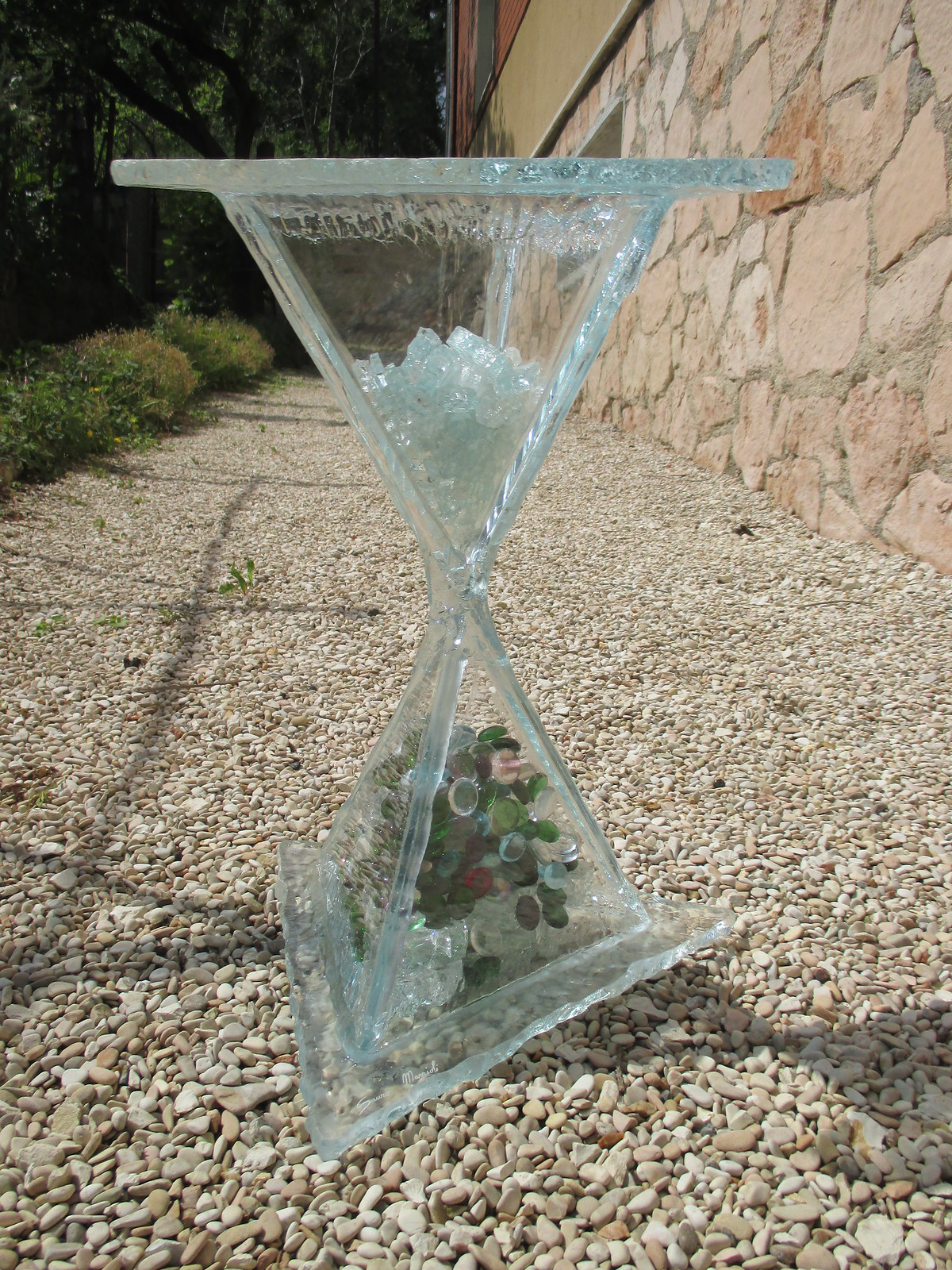The image showcases an outdoor scene featuring an intricate ice-like or glass sculpture that resembles an hourglass. This elaborate art piece is constructed with two triangular prisms, their tips meeting in the middle, creating a clear hourglass shape. The sculpture integrates rough-edged triangular slabs at both the top and bottom, adding to its unique form. The upper section contains transparent crystal-like stones, while the lower section is filled with smooth, round pebbles in shades of green, tan, and red. The sculpture is positioned on a white and tan pebble stone pathway, flanked by greenery including bushes and trees on the left, and a large, light reddish-tan cobblestone wall on the right, suggesting it is in a rustic, outdoor setting. The scale of the sculpture is difficult to ascertain, but it could be as tall as two to three feet.